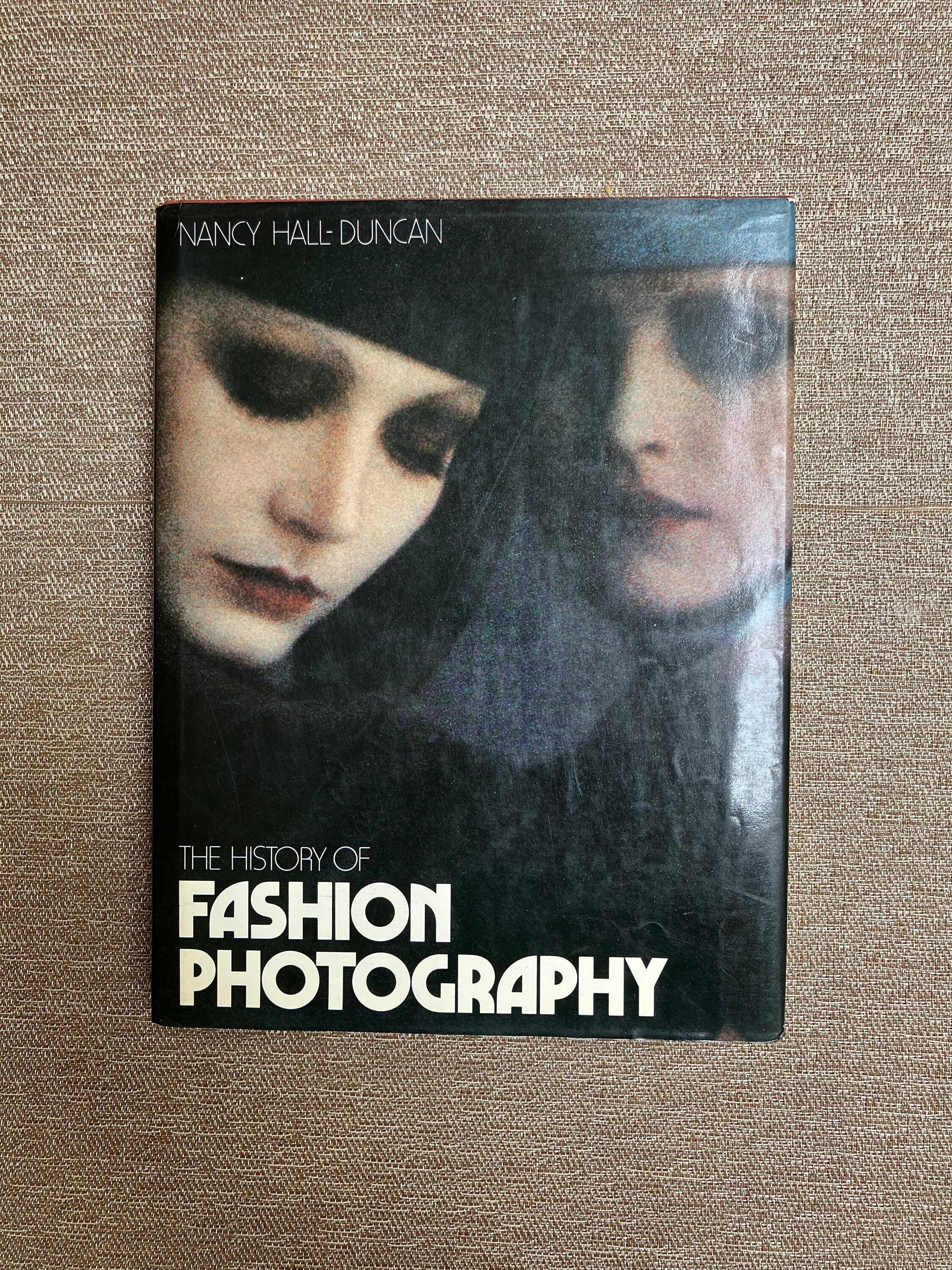Set against a copper-colored, tweed-like fabric that appears soft and speckled with brown, reddish, and white hues lies a glossy hardcover book. The book, adorned with a reflective dust jacket, is authored by Nancy Hall Duncan, as denoted in the upper left-hand corner. Titled "The History of Fashion Photography," the text is prominently displayed at the bottom, with "fashion photography" in large, bold white letters.

The cover features an evocative image of two women with their heads closely wrapped in pillbox-style headgear, which transitions into veils hanging below their chins. Their headscarves come in contrasting colors—one is dressed in black and the other in grey. The background of the photograph is also grey, lending a moody and artsy aura to the image. Their skin appears strikingly pale, which contrasts sharply with their makeup: both exhibit heavily made-up eyes and lips, with dark eyeshadow and vibrant red lipstick.

One woman, dressed in black, is portrayed looking downward with closed eyes, accented by thick black eyeshadow and mascara. The second woman, dressed in grey, is also looking down, with grey eyeshadow that complements her attire. The overall composition exudes a gothic and somber elegance, capturing the essence of high fashion meticulously.